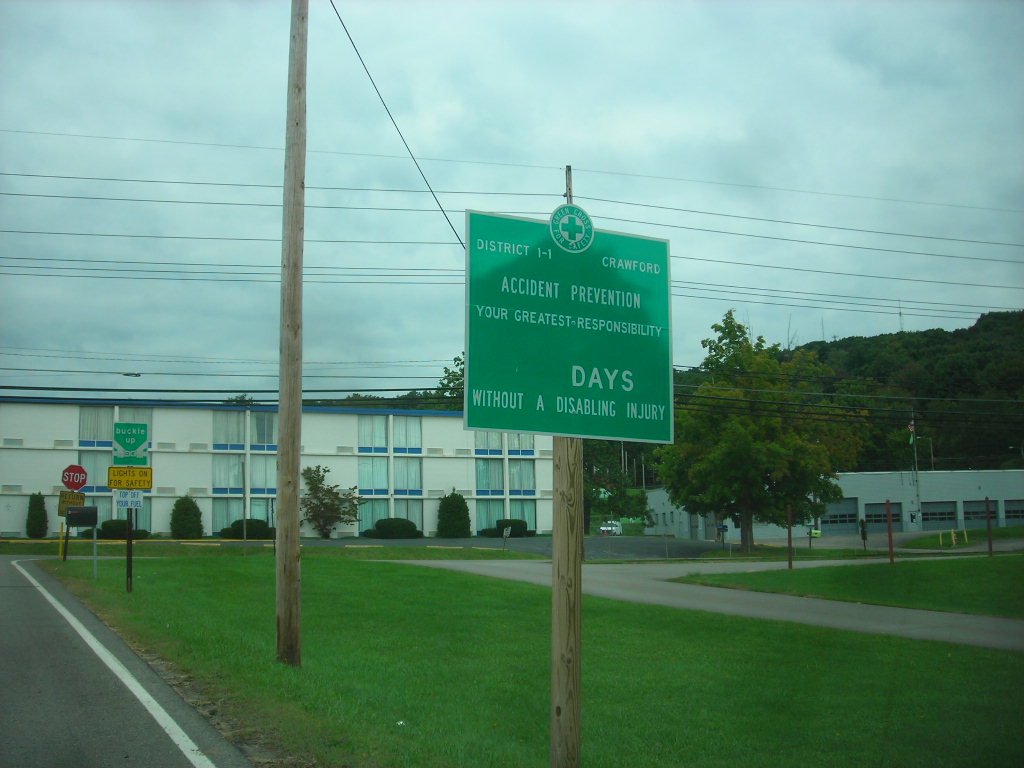In this image, we see a detailed streetscape featuring a combination of signage, buildings, and electrical infrastructure. Off to the left is a grayish road marked with a white stripe. To the right, green grass and a tree adorn the scene, alongside a hill covered with greenery. Electrical wires stretch across the area, supported by a brown wooden electrical pole situated centrally. 

In the foreground, prominently displayed on a square pole in a grassy green area, is a green sign that reads "District 1-1 Crawford Accident Prevention Your Greatest Responsibility Blank Days Without a Disabling Injury," crowned with a green cross symbol. Behind this sign, a red stop sign stands, with additional signs for "Buckle Up" featuring a seatbelt image, "Lights On For Safety" on a yellow background, and "Top Off Your Fuel" in blue letters on a white background.

On the opposite side of the street, there's a three-story off-white building, possibly a hotel, with long windows arranged in columns. Adjacent to this building, to the right, stands a darker gray structure with five garage doors, each fitted with windows. A grayish L-shaped pathway extends towards the right from the green grassy area. At the far end, a black mailbox is visible. The entire scene is framed by additional smaller signs and, in the background, a yellow sign further emphasizing the importance of safety.